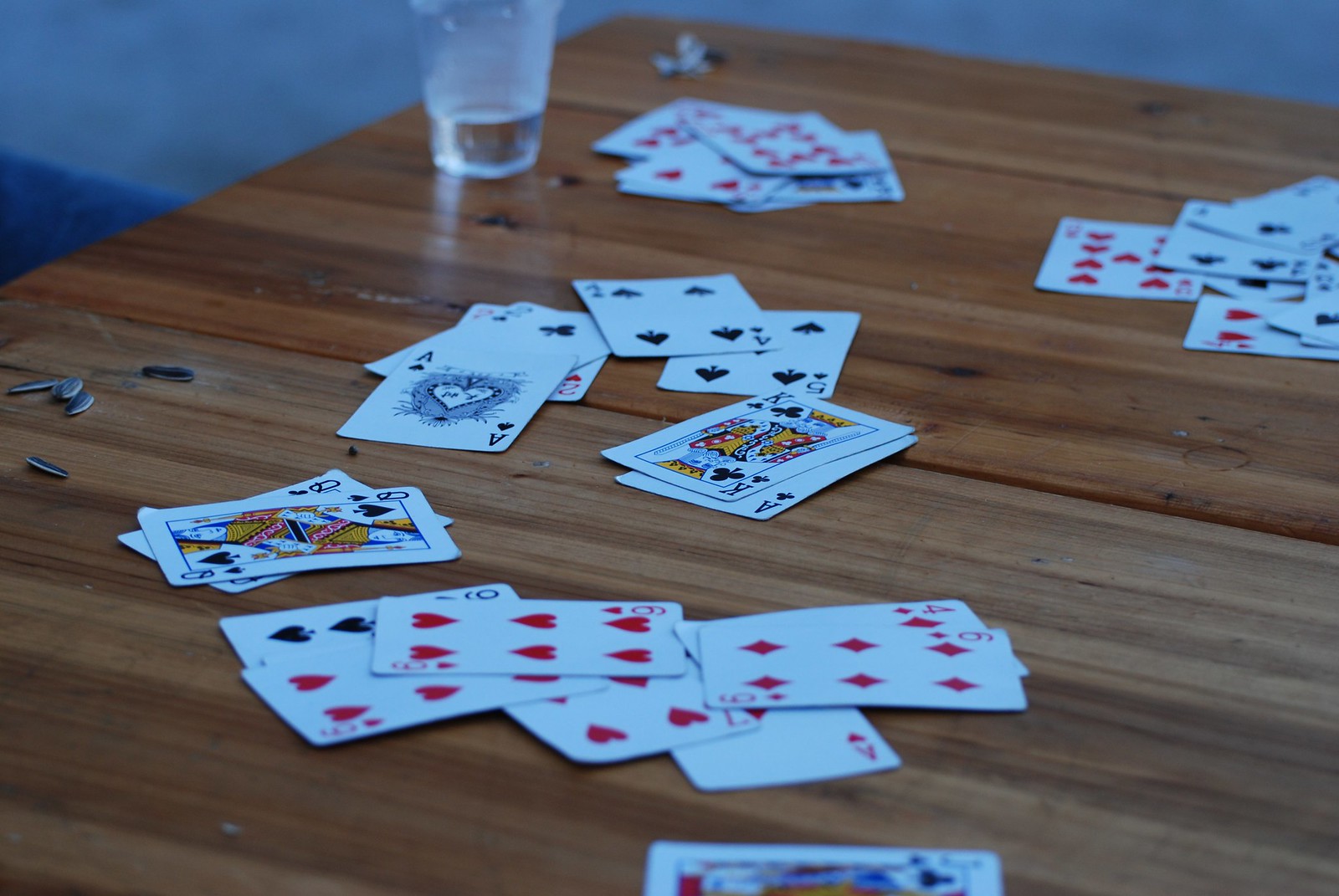In the center of this photograph, a rustic brown wooden table composed of slats dominates approximately 85-88% of the image. The top left and right edges of the table are visible, with its corner positioned near the middle of the frame. Scattered chaotically across the table, a plethora of playing cards create a mosaic of reds, blacks, and whites. 

Towards the bottom of the table lies a Jack of Clubs, while directly above it, a mixture of red cards includes the Four of Diamonds, Six of Diamonds, Ace of Hearts, Seven of Hearts, and two Sixes of Hearts—the latter partially concealing a Nine of Spades. Shifting to the right and slightly upward, two Queens (Queen of Spades on top, Queen of Clubs underneath) rest together.

A secondary cluster of cards—mainly black—features an Ace of Spades overlapping a Two of Clubs, which in turn rests atop a Two of Hearts. This progression continues with a Four of Spades, beneath which lies a Five of Spades. Nearby, a King of Clubs and what appears to be another Ace of Spades or an Ace of Spades-covering the same card are positioned together.

Near the top right corner of the table, a clear glass or plastic cup, quarter-filled with water or another liquid, is close to the edge. Adjacent to this cup is another grouping of blurred cards, the topmost of which is a Ten of Hearts. Slightly left of this arrangement, the Two of Clubs and a Four of Clubs make an appearance, followed by a Nine of Hearts and a Four of Hearts, with a few indistinct cards near the top of the pile.

Lastly, three small metallic objects are discreetly placed at the far right end of the table, adding a touch of intrigue to the chaotic elegance of the scenario.